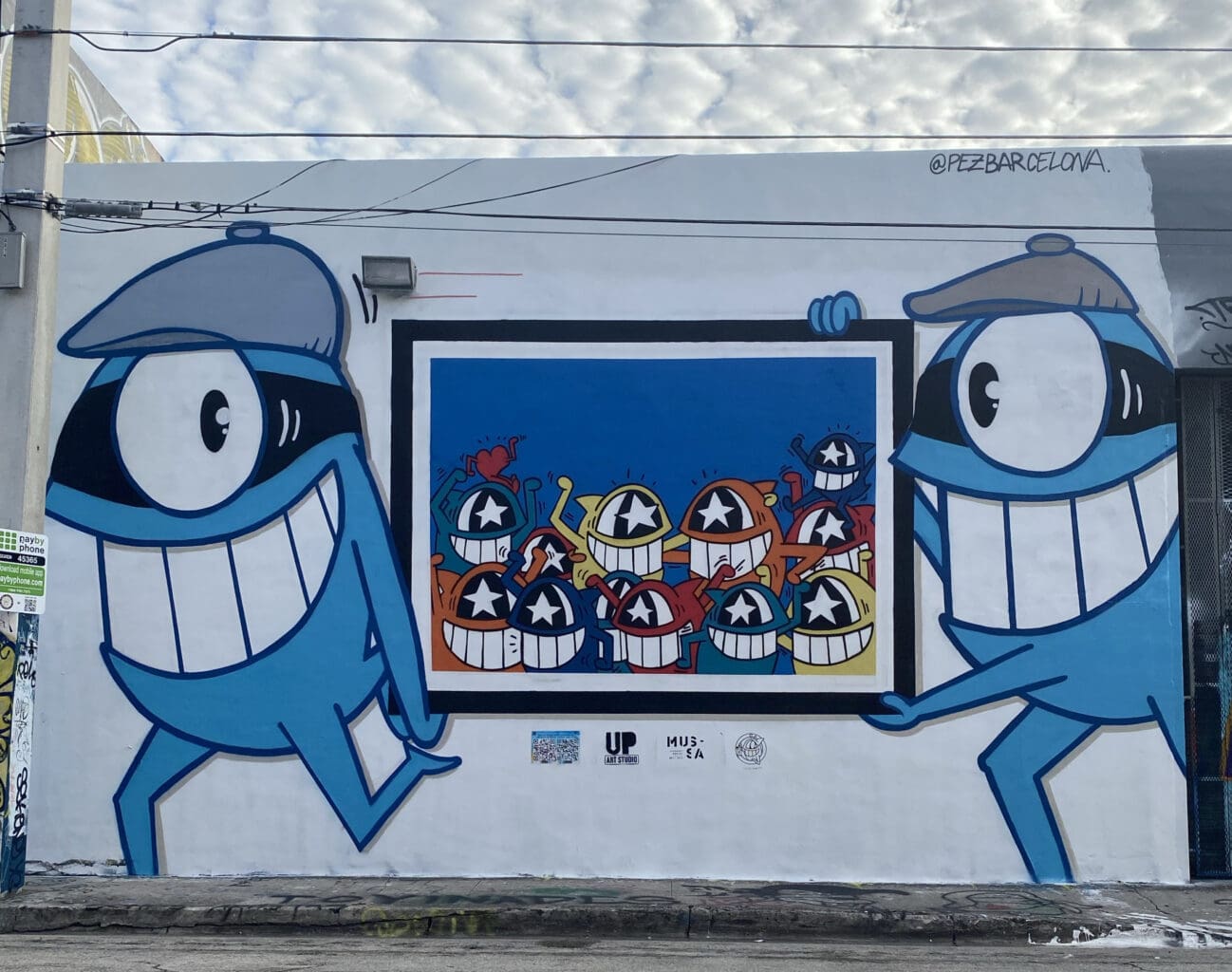The image depicts a vibrant mural on the side of a white building, showcasing two cartoonish, blue alien creatures. These creatures have one large cyclopean eye, big toothy grins, and wear small gray berets. They appear to be in motion, running to the left side of the building, and are each holding one end of a large picture frame. The frame contains a lively illustration of similar alien creatures in various colors—blue, purple, yellow, red—each with star-shaped eyes, hugging and smiling. The mural features a distinctive signature at the top right that reads "@PEZBARCELONA". Above the building, the sky is a deep blue with fluffy clouds, and power lines stretch across the upper part of the scene. At the base, the pavement is gray and cracked.